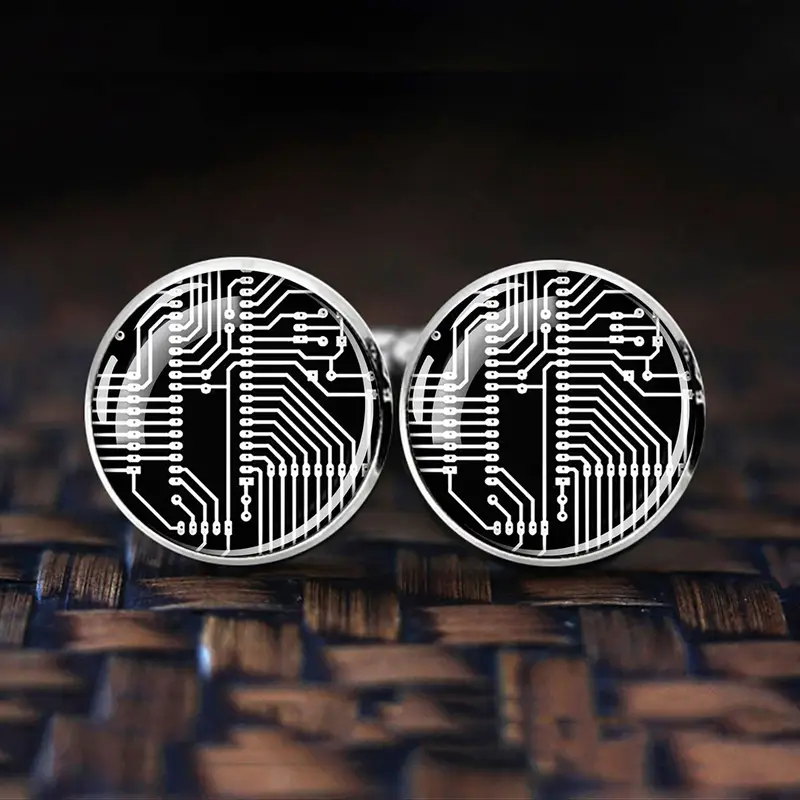The image depicts two round circuit boards placed side by side, each with a metallic silver outline that gives them a sleek, high-tech appearance. The boards showcase intricate white circuit traces, punctuated by black dots resembling solder points, which likely mark positions for electronic components such as IC chips, resistors, and capacitors. A clear glass-like covering on each board suggests a polished, protective layer, evidenced by the visible reflections. The backdrop consists of a woven, wicker-like mat in a natural brown hue, giving the image a contrasting blend of technological and organic elements. The woven texture of the mat appears glossy and fades into the background, adding depth to the composition.